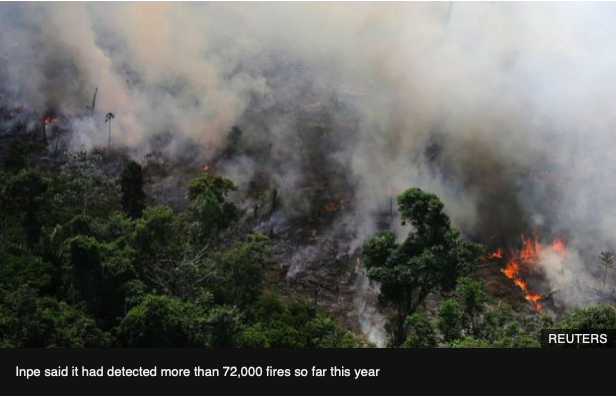This aerial photograph, taken by Reuters, depicts a devastating forest fire engulfing a lush, jungle-like environment. The lower half of the image shows green trees, but the situation quickly deteriorates as the scene transitions to the top half where thick, billowing brown, gray, and white smoke dominates the sky. In the right section of the photo, intense orange flames are clearly visible, rapidly consuming the forest. The pervasive smoke creates a hazy atmosphere with yellow and gray clouds enveloping the area. In the bottom right corner, the photo is credited to Reuters, and a black bar with white text spans the bottom of the image. The text reads, "NP said it had detected more than 72,000 fires so far this year," indicating the alarming frequency of such events.